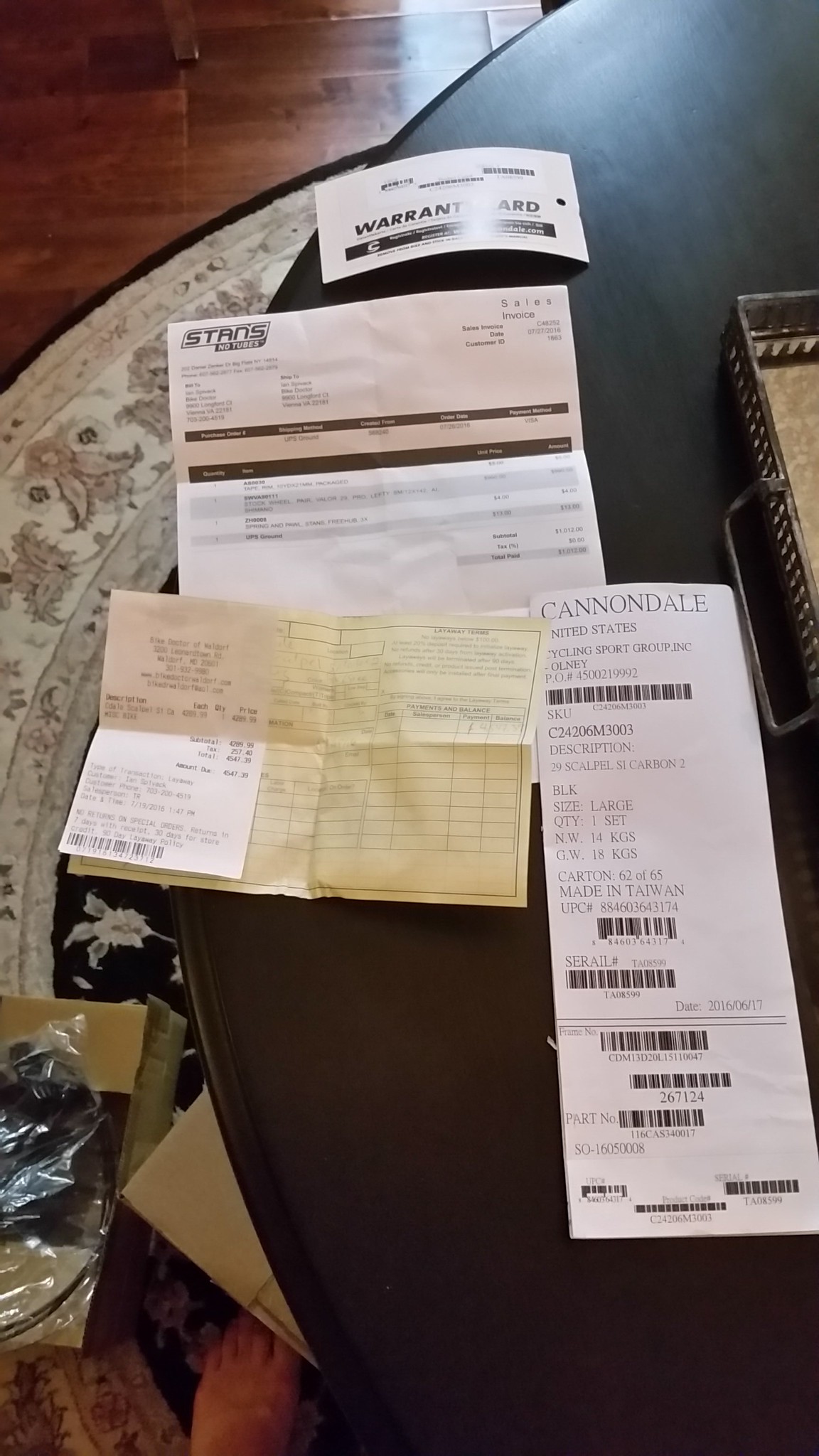In a cozy corner of someone's home, a black round table is meticulously spread out with an assortment of documents. Dominating the scene are four sheets of paper, presumably related to car maintenance. Among them is a visible warranty card placed at the top, and below it, a handwritten yellow carbon copy receipt, complete with a small white receipt stapled to it. An intriguing document marked with "stands, no tubes" and a larger paper labeled "Cannondale United States Cycling Sport Group, Inc." catch the eye. Unintentionally, a person's bare foot is captured in the bottom left corner of the photo. Nearby, two boxes rest on the ground, adjacent to a matching circular carpet that is laid over a stretch of darker mahogany wood flooring, adding a rich texture and depth to the setting.